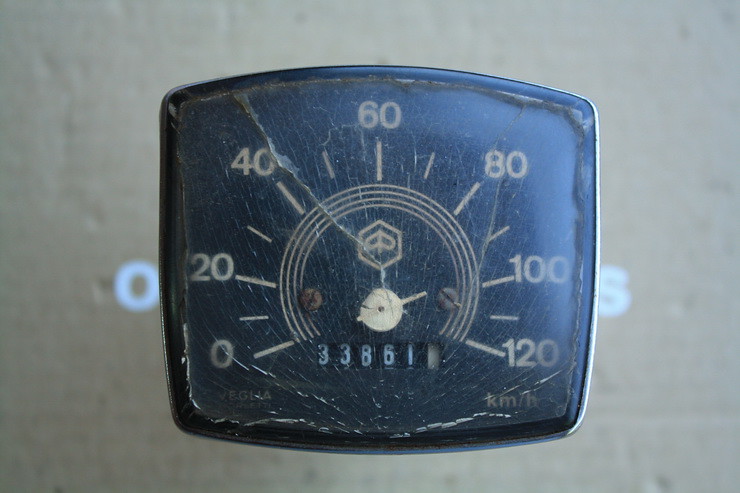This photograph depicts a vintage car speedometer, likely from the 1950s or 1960s. The speedometer's housing is a somewhat rectangular shape with subtly curved edges, enclosed by a plastic cover that shows significant wear. A prominent crack runs diagonally from approximately the top left corner to the center, with additional shards and fractures particularly visible around the edges. The dial itself features four concentric circles, intricately printed, forming the graduated measurement lines.

The speed indicator needle is notably short and may be broken, which could affect its ability to accurately point to the recorded speeds. The speed scale, measured in kilometres per hour, ranges from 0 up to 120, marked in increments of 20. On the bottom right-hand side of the dial, the abbreviation "km/h" confirms the unit of measurement. Additionally, an odometer displays the vehicle’s total distance travelled, reading 33,861 kilometres. The overall condition of the speedometer, including the cracked plastic and potentially damaged needle, suggests it has seen considerable use over decades.